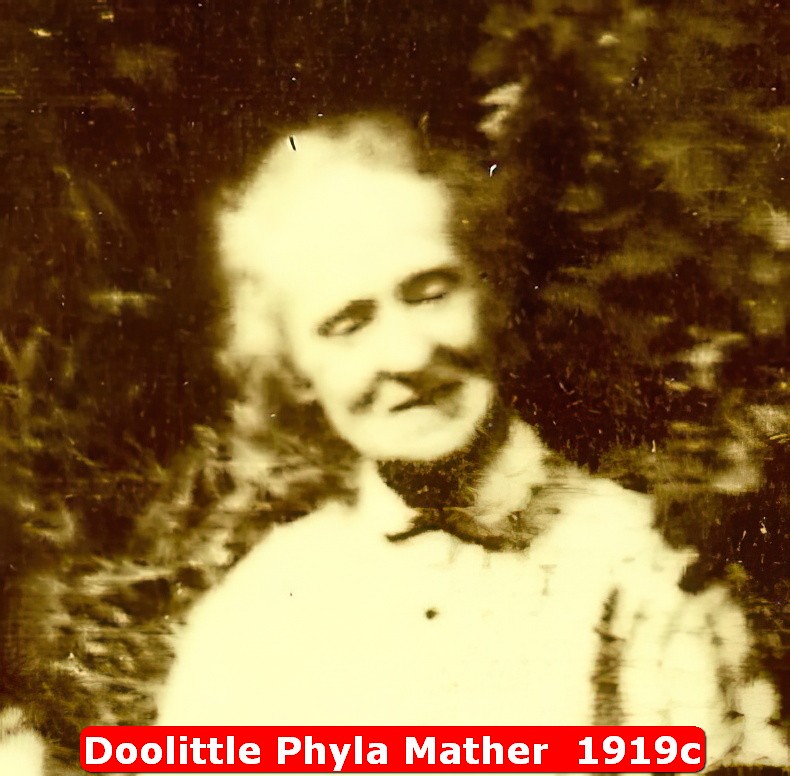This image is an old, black and white or sepia-toned photograph, possibly of poor quality or faded over time, appearing to have been scanned onto a computer. It features an older person, very likely a woman given her name, Phyla Mather, written in white letters on a red banner located at the bottom of the image, reading, "Doolittle Phyla Mather, 1919 C." The photograph is not in great focus and shows numerous imperfections and niches. The woman, who appears to have slightly long, grayish hair reminiscent of Einstein’s, is wearing a light-colored collared shirt or dress that ties tightly at the neck. Her head is cocked slightly to her left (our right) and she is posed in front of indistinct greenery, perhaps bushes or trees. The photo is cropped at chest level, with her left arm and shoulder visible in the bottom right corner, positioned against a backdrop of brush and tree limbs to the left and right of her. Overall, the quality of the image makes it hard to discern specific details clearly.